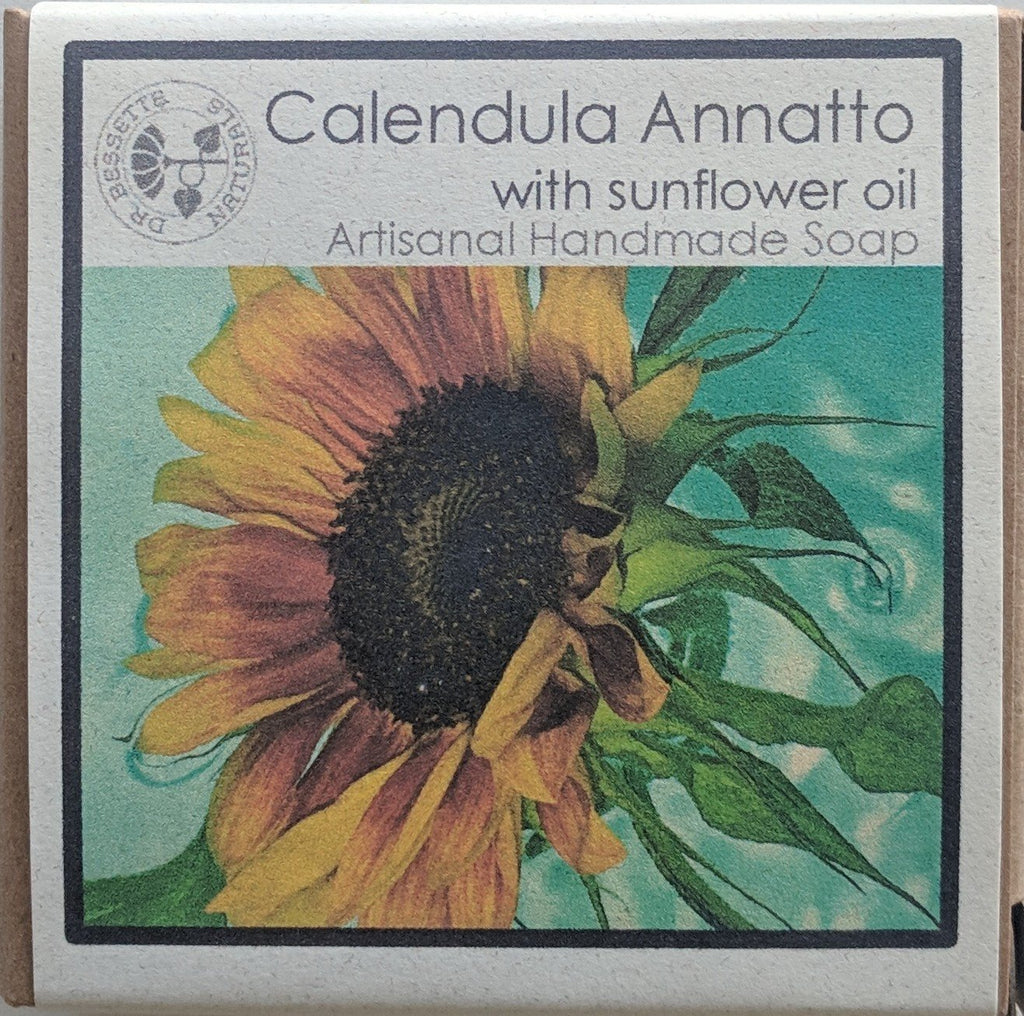The image showcases the outer packaging of an artisanal handmade soap. The label is printed on a piece of off-white, recycled-quality paper with a thin black line border and is glued to a rustic brown box. At the top of the label, in black lettering, it reads: "Calendula Annatto with Sunflower Oil, Artisanal Handmade Soap." Below the text, there is a detailed and colorful drawing of a sunflower. The sunflower features vivid yellow and reddish-orange petals surrounding a dark brown center, with visible seeds and some open cavities. The sunflower also has dark green leaves, set against a background of greenish-blue sky with white clouds. The paper edges are brown, mimicking the look and texture of cardboard, which adds to the artisanal aesthetic of the packaging.